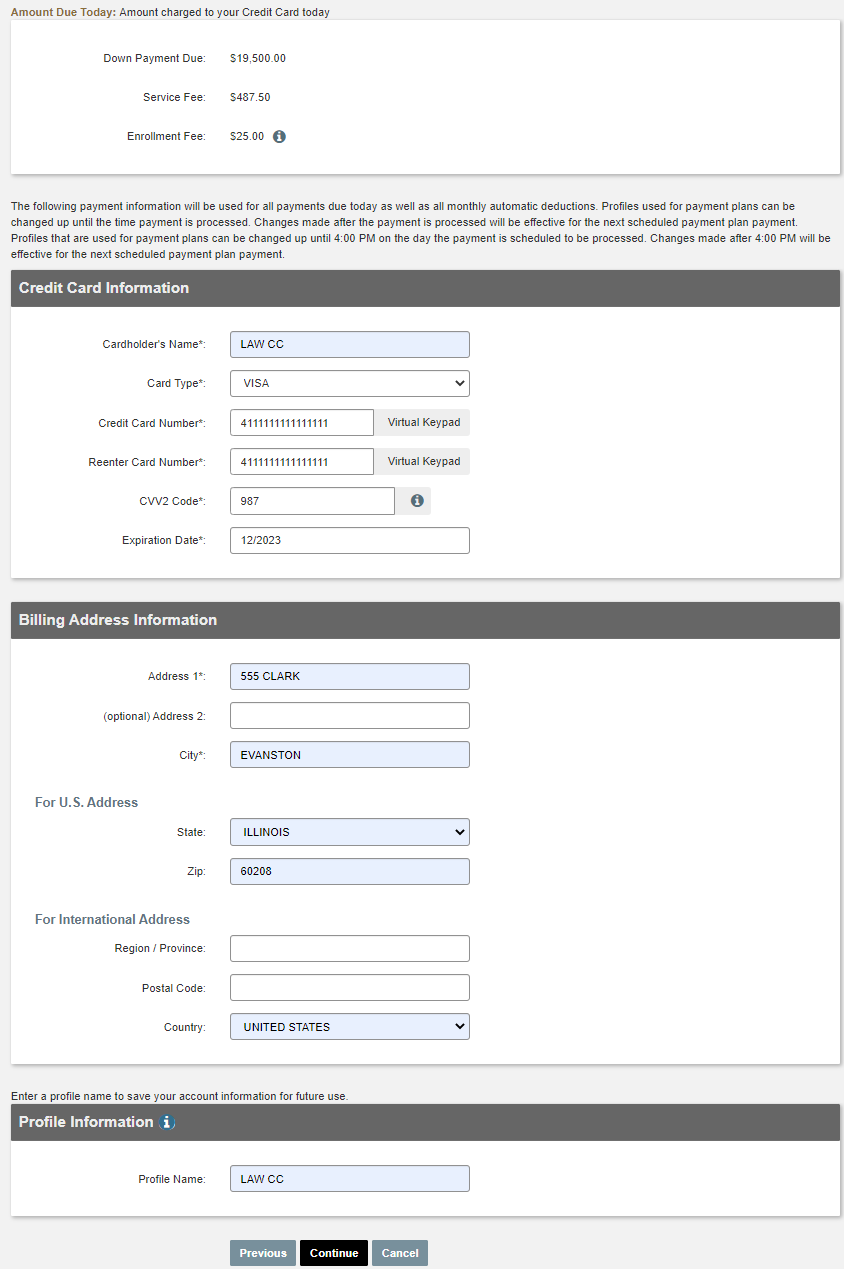At the top of the image, there is a white area featuring a header with three lines of text, which are mostly unreadable. Below this section, a gray background contains a paragraph filled with text. Beneath the paragraph, there is a black box labeled "Credit Card Information" that includes a column on the left with various labels and six text input boxes on the right. Following this, another black box labeled "Billing Address Information" is present. It has three input boxes at the top, with a note indicating "for U.S. address," one of which is labeled "State" with "Illinois" filled in and another labeled "Zip Code." Below these, there are three additional boxes designated for international addresses. At the very bottom of the image, there are three buttons: a blue button on the left, a blue button on the right, and a black button in the middle.